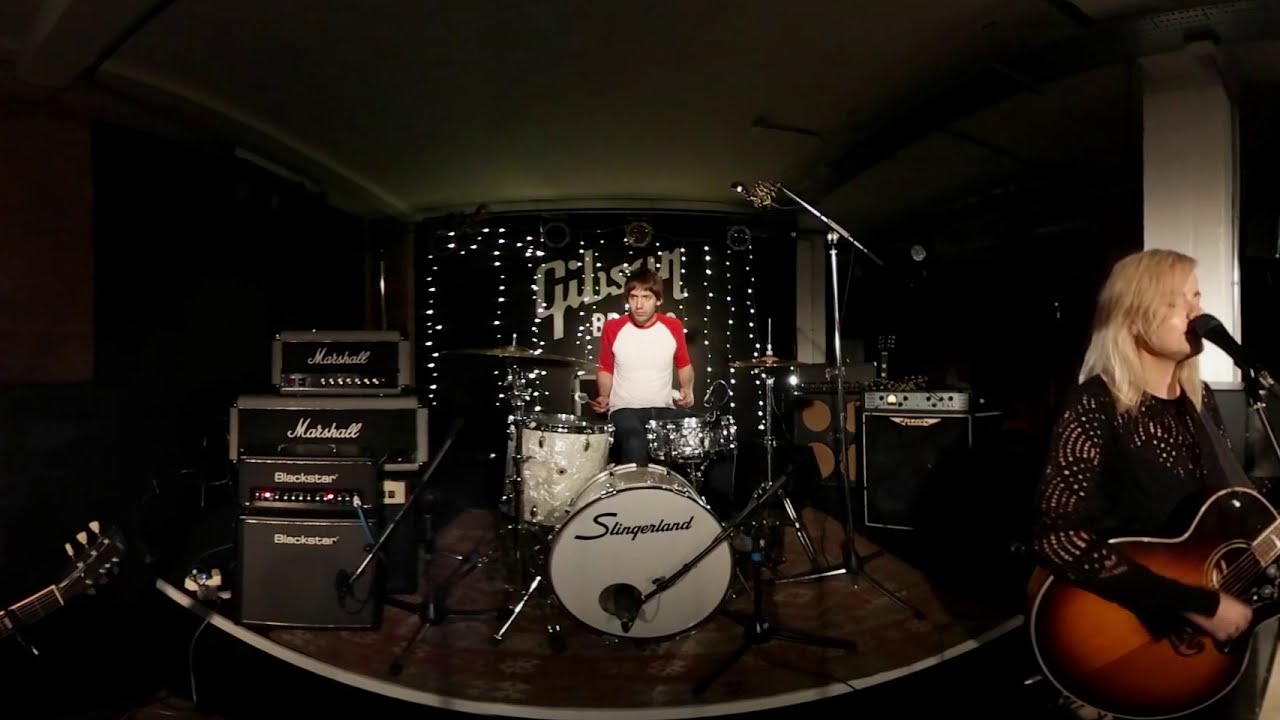The image captures an indoor stage scene with a musical band actively performing. Central to the image is a drummer, a Caucasian male with brown hair, dressed in a white shirt with red sleeves. He's engrossed in playing a silver and white Slingerland drum set. In front of him, towards the right-hand corner, stands a female guitarist with blonde hair, also Caucasian. She is wearing a black long-sleeved blouse and appears to be energetically strumming an acoustic guitar while singing. The stage, which has a low brown wooden platform, is adorned with a plethora of musical equipment including multiple amplifiers from brands like Marshall and Blackstar. The backdrop features the word "Gibson" illuminated by Christmas lights, adding a festive ambiance. A third band member, partially visible on the left side of the frame, is playing another guitar, although only the neck of the guitar is discernible. The overall setup conveys a well-equipped band either practicing or performing, with detailed attention to musical gear and atmospheric stage lighting.